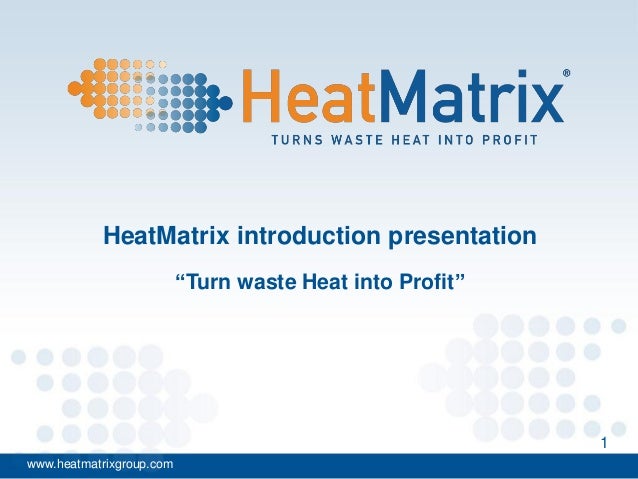The image is a professional slide designed for a PowerPoint presentation for a company called Heat Matrix®. The background at the top of the slide is light blue, featuring a dotted icon that transitions from orange to blue circles. Centered at the top-left corner, the Heat Matrix logo is displayed with "Heat" in orange and "Matrix" in blue as a single word. Adjacent to the logo is the registered trademark symbol (®). Beneath the logo, in smaller navy blue uppercase font, it reads "TURNS WASTE HEAT INTO PROFIT." Below this, in blue text and centered on the slide, it states "Heat Matrix Introduction Presentation," followed by the phrase in quotation marks, "Turn waste heat into profit." The bottom half of the slide has a white background with circle designs on both the left and right sides. At the very bottom, a blue number "1" is positioned in the lower right-hand corner, while the URL www.heatmatrixgroup.com is in small white font on the lower left-hand corner. Noteworthy is a slight inconsistency where the word "waste" is not capitalized in the phrase quotations.